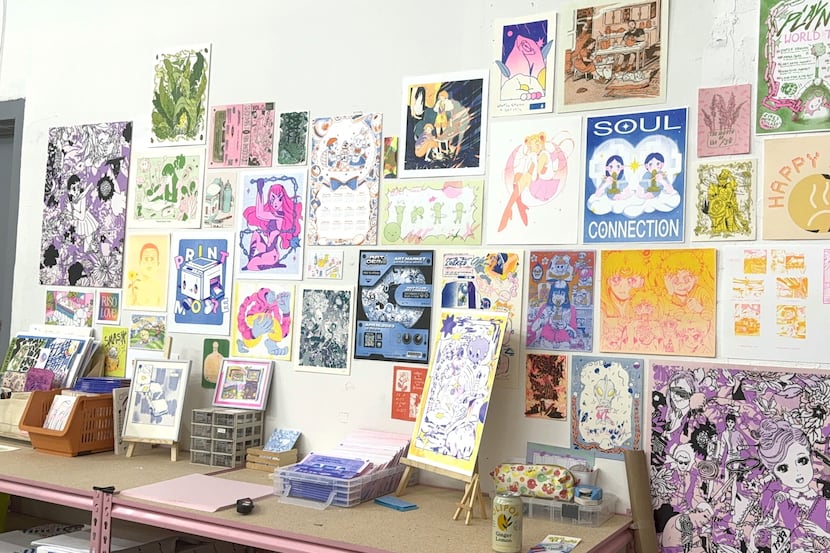The image depicts an arts and crafts corner in a room, featuring a long, rectangular desk made of a thin, particle board and painted pink on the edges. The desk, which is brown aside from its edges, is pushed against a white wall and appears to have shelves underneath, storing various arts and crafts supplies in little plastic containers. On the desk, there are several miniature easels displaying artworks, including one with a yellow frame and a white-blue interior with a few characters. The desk also has a yellow can situated below the central artwork. The white wall in the background is densely covered with small, hand-built-sized artworks, predominantly in anime style with characters that resemble Sailor Moon. The overall color scheme is a mix of yellows, pinks, purples, natural greens, and whites, creating a girly, pastel ambiance.